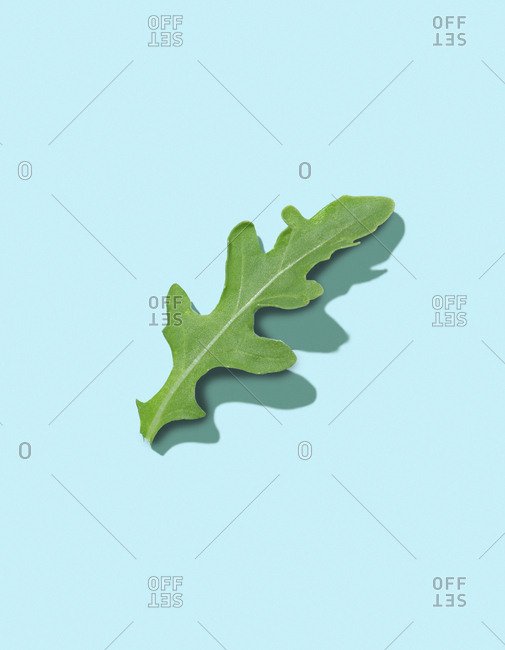A detailed graphic image features a rounded green leaf prominently centered against a light blue, almost turquoise background. The leaf, light green in color with edges that undulate and curve inward and outward, culminates in a rounded tip near the upper right. A prominent white vein runs down the middle, with thinner white veins extending towards the leaf’s edges. The surface on which the leaf rests casts a noticeable shadow, adding depth to the image.

Overlaying the entire scene are faint, grid-like lines that give the background a paper-like texture. Superimposed on both the leaf and the background are repetitive text elements: “0,” “OFFSET,” and “SET,” with “SET” appearing backwards. These words, designed in varying shades of gray and white, are angled and likely serve as a watermark to prevent unauthorized use of the image. The overall composition—with its graph paper undertones, watermark text, and detailed leaf veining—creates a visually interesting and complex graphic.